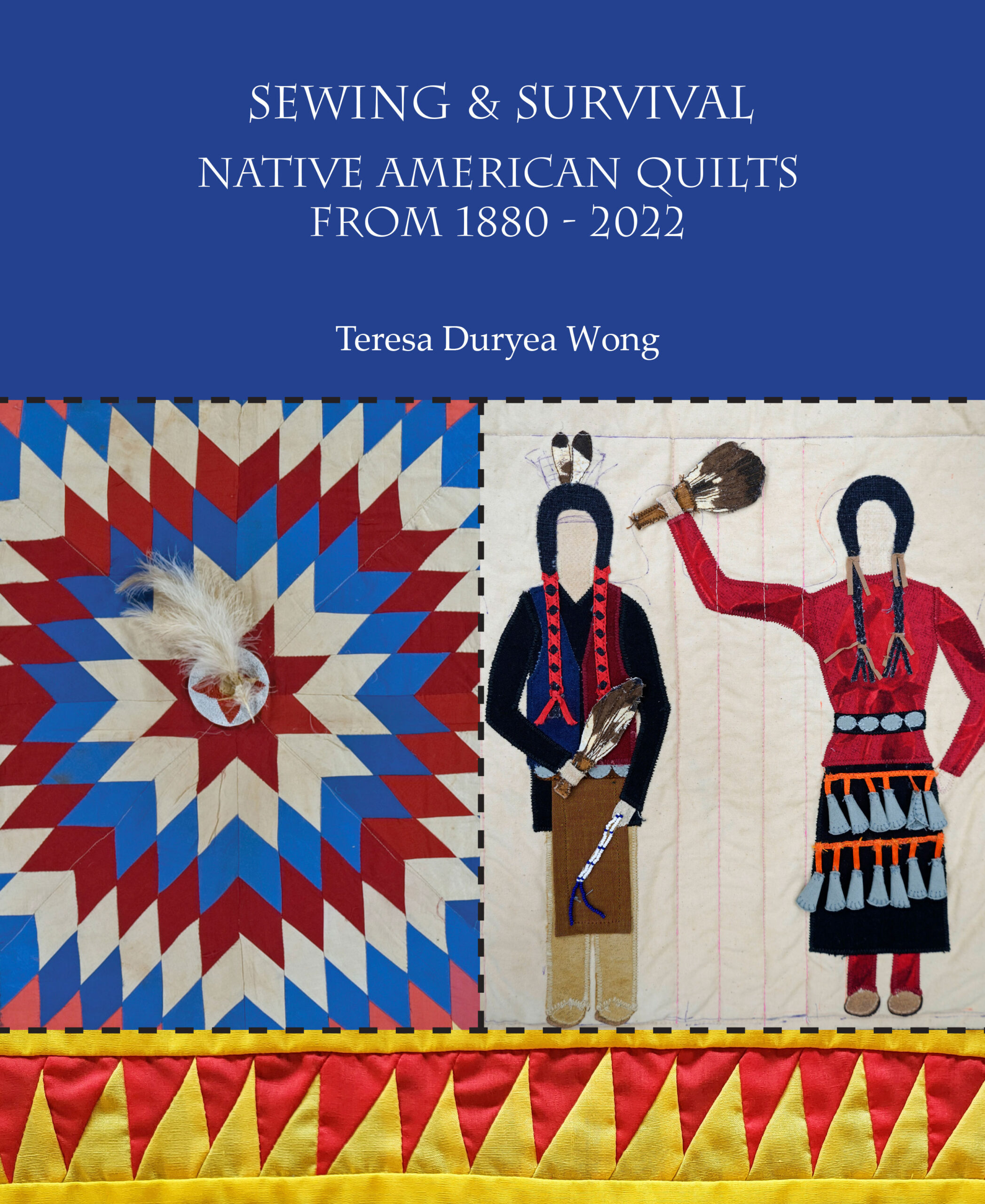The image is a highly detailed poster or book cover. At the top, there is a vivid blue rectangle spanning from left to right, with the text "Sewing and Survival, Native American Quilts from 1880 to 2022, Teresa Duryee Wong" prominently displayed in white, likely in a Times New Roman font. Beneath this text section, a black dashed line runs horizontally, mirroring another dashed line dividing the page vertically into two halves.

On the left side of the vertical dashed line, there is a colorful quilt featuring a central feather motif surrounded by a star pattern. The quilt's design alternates in red, white, and blue layers, creating a striking geometric form.

To the right of the vertical dashed line, there is an illustration depicting two Native Americans in traditional attire. One figure, possibly male, has long braided hair adorned with feathers, wears a blue and black top, and a brown apron. The other figure, likely female, also has long braids adorned with tan tassels, a red shirt, a belt with blue dots, and a black skirt with orange horizontal lines and blue tassels at the ends.

At the very bottom, another horizontal black dashed line separates the main content from a bottom section that features a yellow background adorned with downward-facing red triangles, resembling flags or decorative embellishments. This intricate design integrates cultural elements and textile art, capturing the essence of Native American quilting traditions.